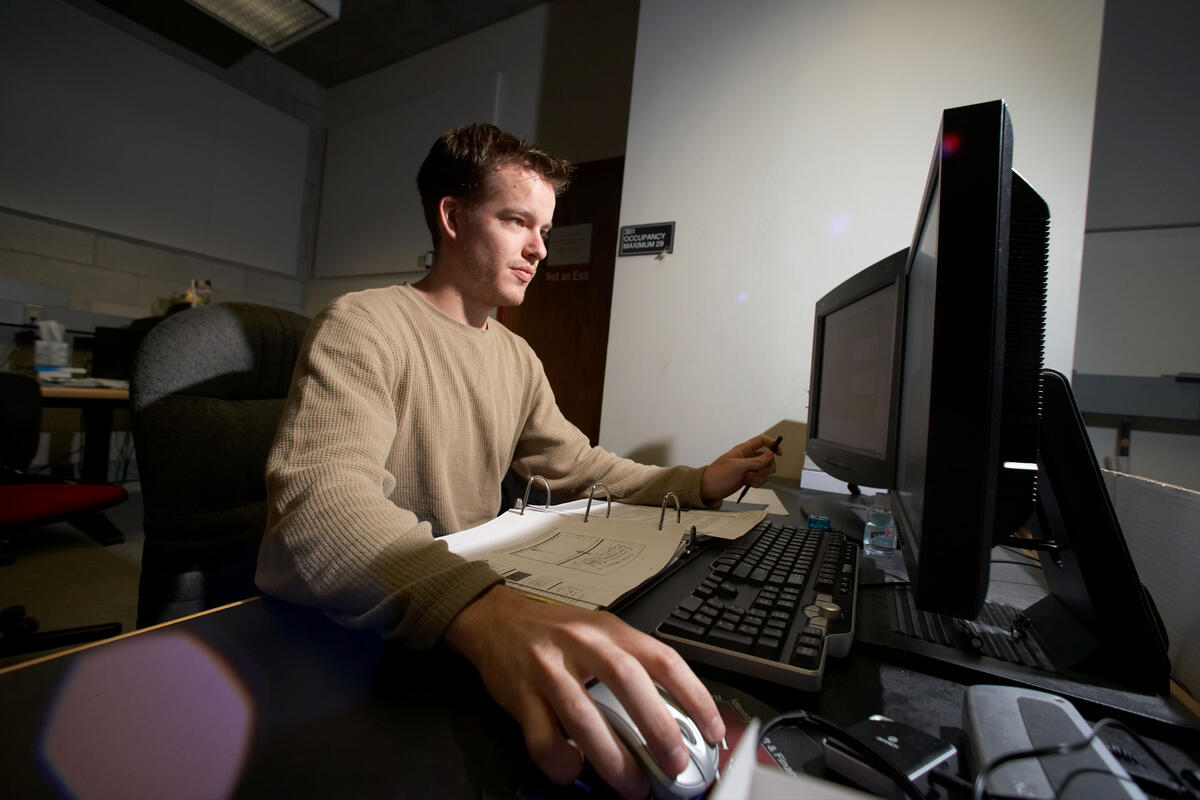The image portrays a young man, possibly in his early twenties, focused intently on his work at a desk in a professional office or workspace setting. He has short, dark brown hair and is clad in a long-sleeve, grayish-tan sweater. Seated in a gray chair, he commands a dual-monitor computer setup, with his right hand positioned on a mouse and his left hand holding a pen or pencil. The desk, which has a dark or purple-hued surface, supports a keyboard and an open three-ring binder filled with papers. The man, whose expression ranges between serious concentration and a slight smile, appears to be deeply engaged with the content on the main monitor. Behind him, the room extends with another desk and chairs, suggesting a shared workspace. The background features a white wall, partially adorned with a black plaque, and the overall lighting is somewhat dim, augmented by subtle fluorescent lights above, indicating a typical office environment.